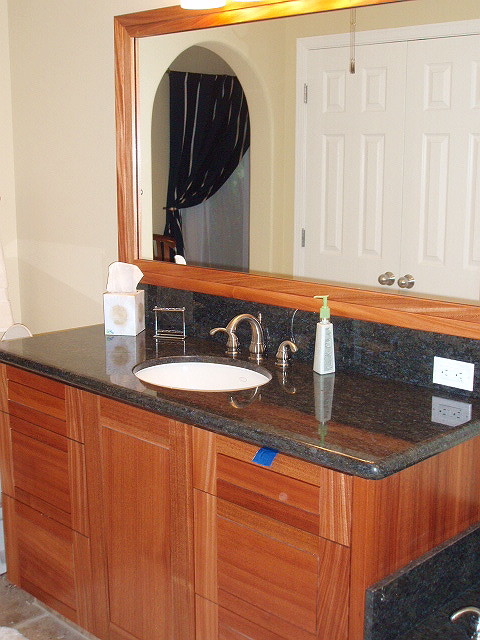This photo captures a well-appointed bathroom with a detailed view of the vanity area. The countertop is a dark granite, presenting a sleek and elegant look. Set into the countertop is a single sink, featuring a bronze faucet head with matching hot and cold taps on either side. To the left of the sink, there is a white tissue box, accompanied by an empty, square, metallic soap holder.

On the right side of the sink rests a flat, green soap pump bottle. Additionally, a white, square electrical plug is visible against the granite surface. 

The vanity below the countertop is constructed from dark wood, with functional metal cabinet handles and several drawers for storage. Above the sink, a large mirror framed in the same dark wood as the vanity creates a cohesive design, and it is accentuated by a light bar mounted directly above, providing ample illumination. The overall aesthetic of the bathroom exudes both functionality and sophistication.